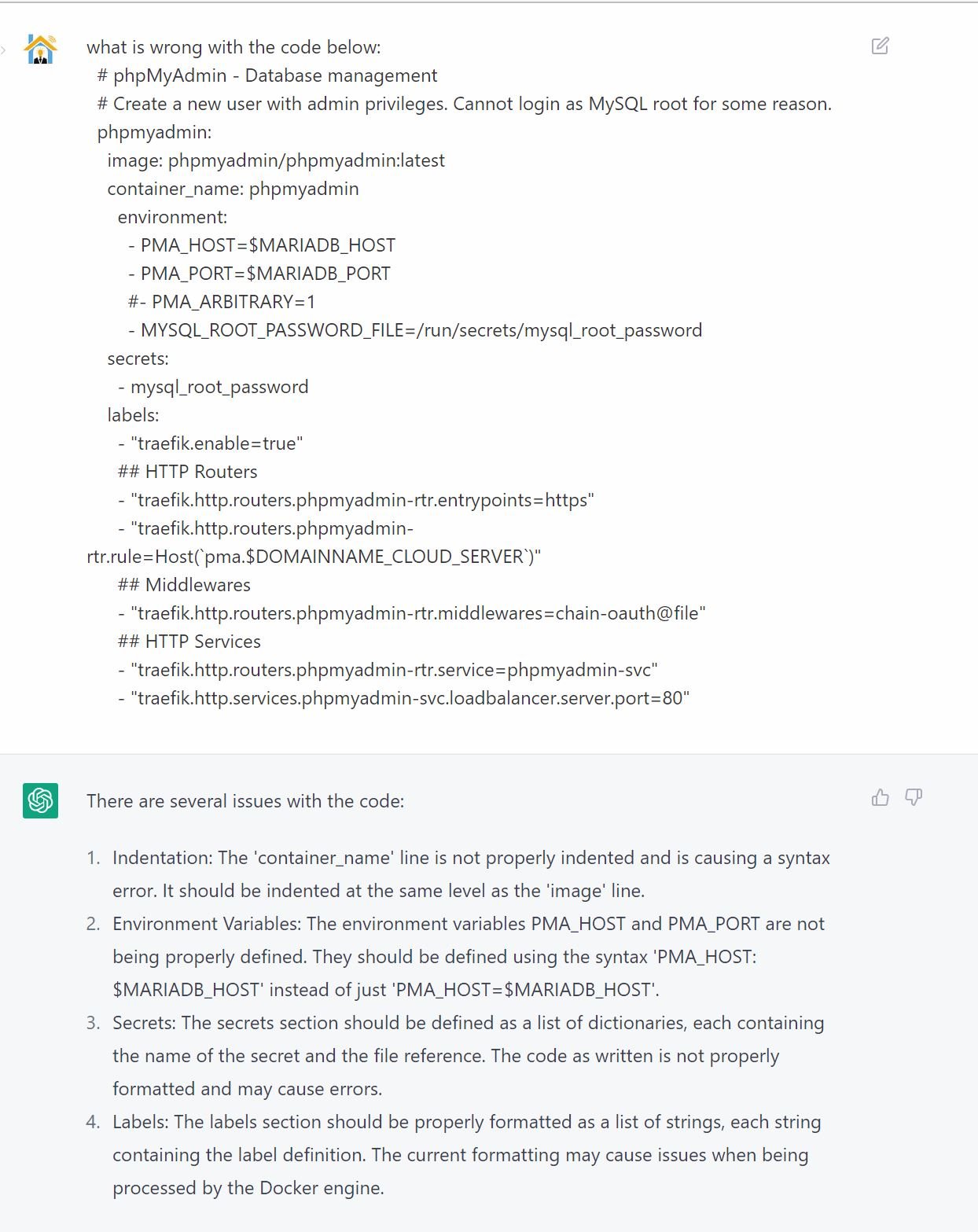A screenshot from a website showcasing a ChatGPT interface. At the top, the user's message appears, asking "What is wrong with the code below?" followed by a snippet of code starting with the comment `# phpmyadmin-databasemanagement`. The code seems to relate to creating a new user with administrative privileges in a MySQL database, though the user mentions they cannot log in as the MySQL root for some reason.

The ChatGPT response is displayed in a darker gray box with black lettering and features the green ChatGPT logo on the left side. The response outlines four main issues with the provided code:

1. **Indentation**: The response describes specific parts of the code where indentation errors are present.
2. **Environment Variables**: It explains that the environment variables are incorrect and need adjustment.
3. **Secrets**: This section should be defined as a list of dictionaries, each containing the name of the secret and the file reference.
4. **Labels**: The labels section must be properly formatted as a list of strings, with each string containing the label definition.

At the top right corner of the ChatGPT response box, there are thumbs up and thumbs down icons for user feedback.